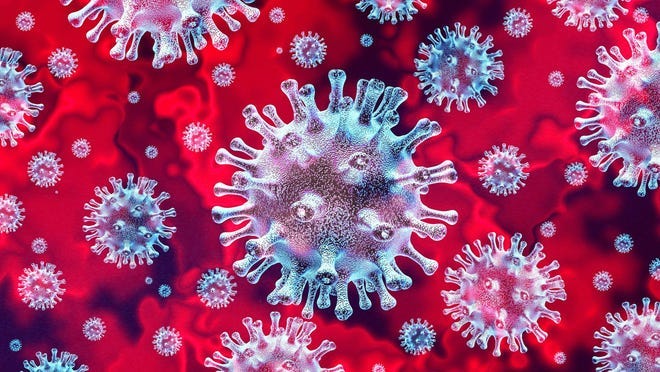The image is a detailed, color illustration depicting what appears to be an artistic rendering of COVID-19 viruses or cellular organisms. The central focus is a large, white, and bluish orb, adorned with numerous protrusions that terminate in small bulges, each featuring a hole at the tip. Surrounding this central figure are dozens of smaller, similarly structured orbs, creating a dense, clustered arrangement. The background is a variegated blend of black, red, and some gray areas, adding a dynamic, almost fluid-like contrast to the white-blue foreground. The illustration, with its non-photorealistic, digital art style, conveys a sense of floating, opaque orbs resembling spike proteins, reminiscent of the coronavirus. The varying sizes of the orbs, larger at the forefront and smaller in the background, enhance the depth and complexity of the scene, capturing the intricate, almost abstract nature of the subject.